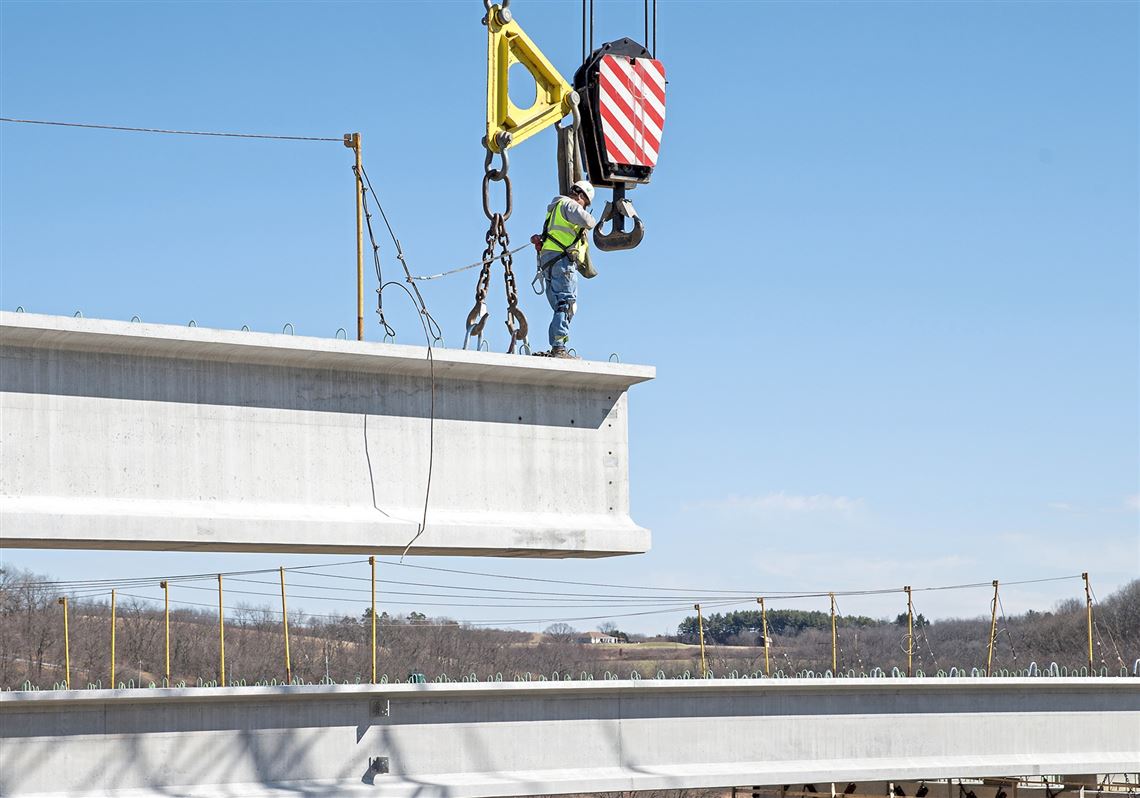In the photograph, a construction worker is standing confidently on the edge of a large, grayish steel I-beam that is suspended in mid-air by thin, black chains connected to yellow crane hooks. The beam, being guided into place, hangs over another I-beam positioned directly below, suggesting ongoing construction at a considerable height. The worker, donning a bright yellow safety vest, blue jeans with knee pads, sturdy boots, and a white helmet, appears to be connecting or adjusting a massive crane hook held in front of him. The expansive background reveals a brownish landscape with scattered tumbleweeds, and a distant house can be seen far off in the horizon, framed by a light blue sky. The scene captures the worker’s calm expertise amidst a precarious, high-altitude task.